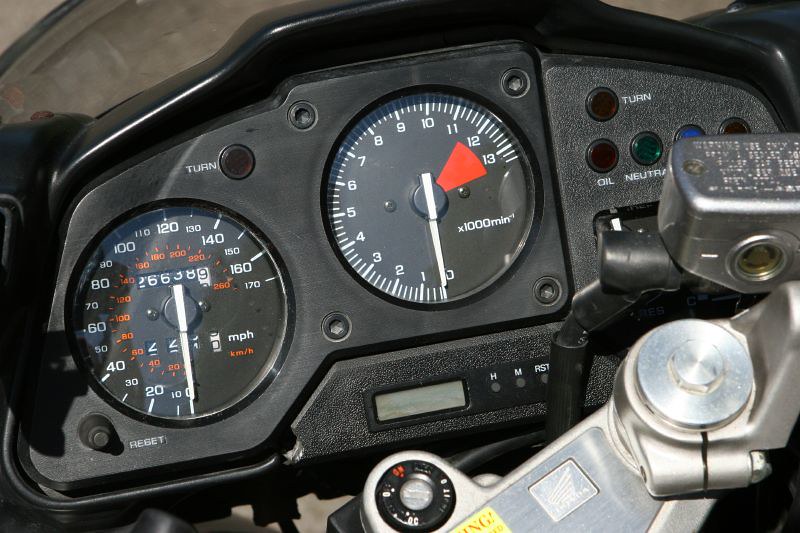This image captures the intricate details of a motorcycle's dashboard and controls. Dominating the top portion of the photograph is a black panel. Centrally located on this panel is a prominent button labeled "TURN" in white text. Adjacent to this is a circular speedometer. The outer ring of the speedometer displays numbers from 0 to 170 in white, while an inner ring lists numbers from 0 to 260 in yellow, denoting the speed in kilometers per hour. Below the speedometer, the total kilometers ridden, 266,389, are displayed in a black and white digital readout, and alongside it, the numbers 220 and the notation "MPH" in white denote the speed in miles per hour, with kilometers indicated in yellow. 

An indicator line is currently positioned at 0. To the right of this main circle, there's an additional gauge that shows numbers ranging from 0 to 13 in white, possibly representing the RPM. Just below this gauge is red text reading "x1000 min^-1" in white, indicating RPM x1000.

Within the dash, an arrangement of indicator lights glows in orange, red, green, and blue, accompanied by a red button labeled "10" in white and an indicator for "NEUTRAL" also in white. Lower on the panel, the words "HM" and "RST" appear in white, likely representing additional settings or reset functions. A silver metallic component, probably part of the ignition system, along with what seems to be the ignition button, is also visible at the bottom of the image.